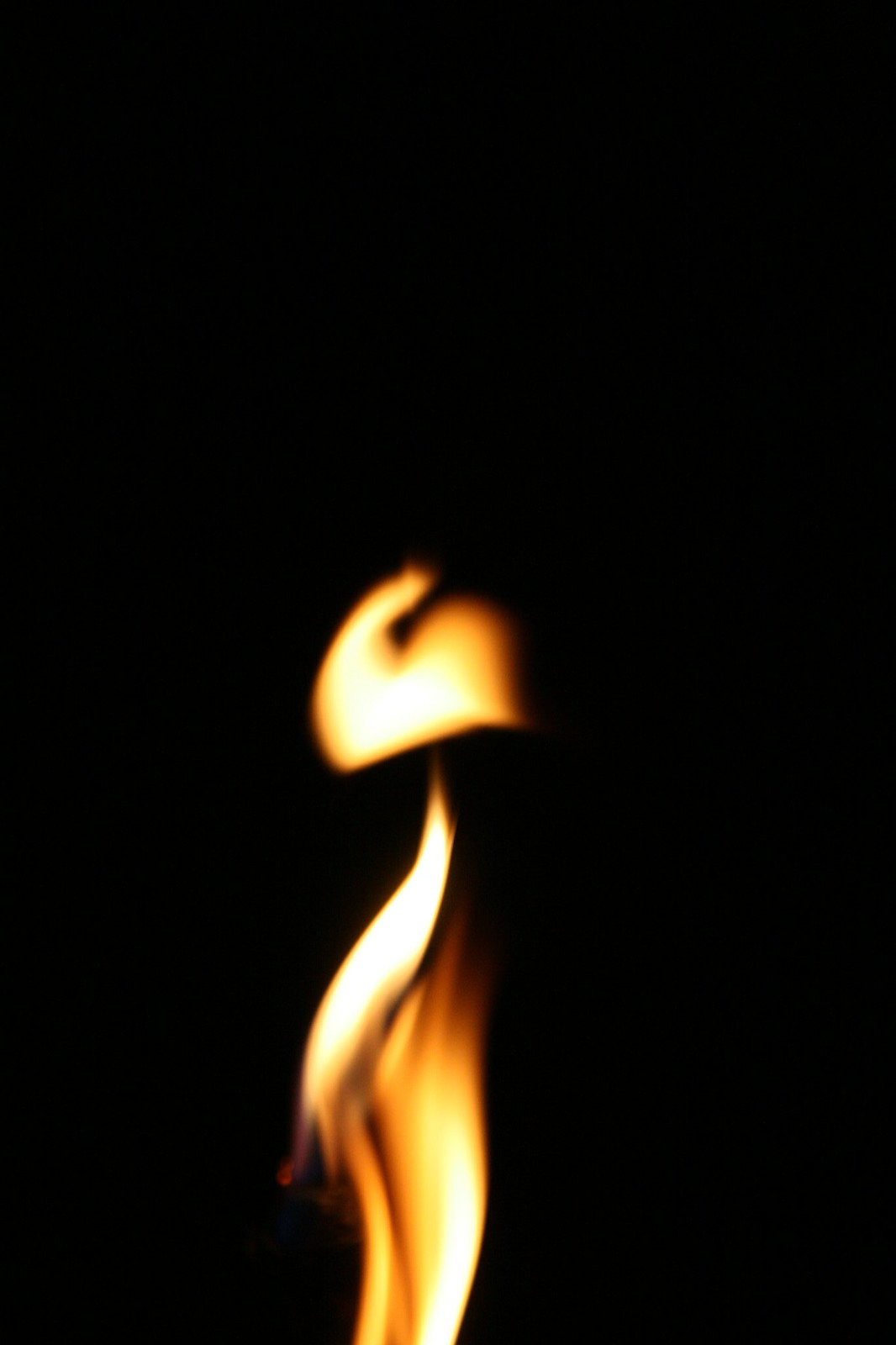This slightly blurred image, set against an entirely black background, captures a vivid depiction of a flame. The flame occupies the center of the image, extending about two-thirds of the way up in a narrow yet dynamic form. It showcases a mesmerizing blend of colors, including bright yellows, deep oranges, and whites, with darker reddish-orange hues accentuating its edges. 

The flame appears to be composed of two distinct parts: the lower section has a flowing, ribbon-like quality that twists and curls, reminiscent of a tapered lily shape. This section displays a rich palette of orange shades, seamlessly transitioning to white at the top. Meanwhile, the upper portion features a half-circular flourish that suggests the tip of a flame stretching upwards. This part includes brighter yellows at its core, bordered by dark orange-red edges.

The interplay of these colors and the intricate shapes within the flame evokes a sense of movement and realism, despite the slight blur that softens its exact details. The photograph's portrait orientation and the detailed abstract representation of the flame make it a striking visual, capturing the essence of a flame in a stylized yet lifelike manner.